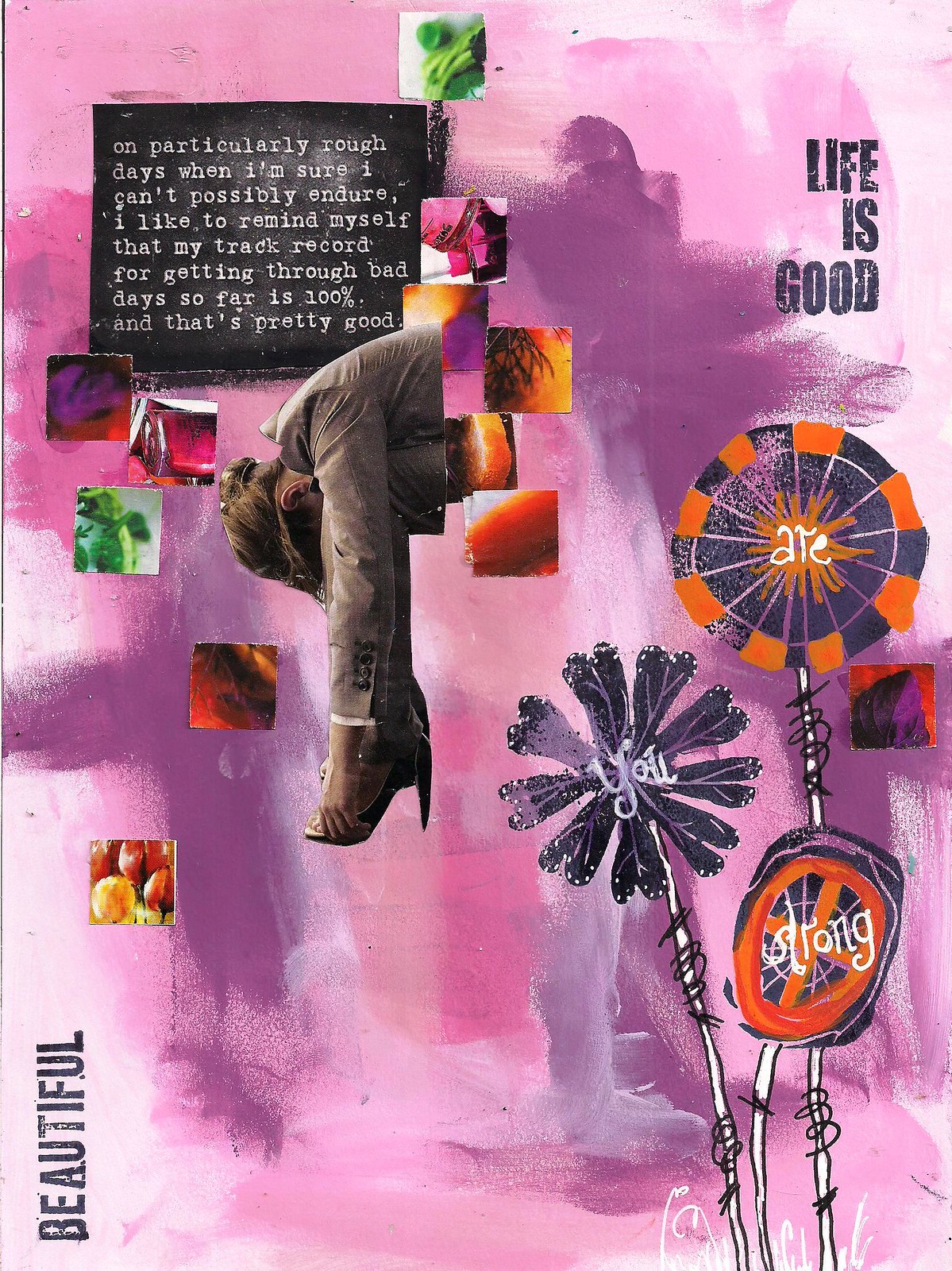The image features an abstract, predominantly purple background with pink and white accents. At the center is the top half of a woman dressed in a suit jacket and high heels. She is bent over, with her head between her knees, appearing as if she has fainted and is trying to get blood back to her head. Her hair is styled in a bun, and the lower half of her body is cut off by the edge of the image.

Surrounding the woman are various colorful squares, some depicting fruits, vegetables, and trees, adding a collage-like effect to the artwork. Among these squares, there's an orange one with what looks like trees and another with tree-like shapes that resemble lollipops.

In the upper left corner, against a black rectangular background, is a motivational quote in white lowercase letters: "on particularly rough days when I'm sure I can't possibly endure, I like to remind myself that my track record for getting through bad days so far is 100%, and that's pretty good." In the upper right corner, the text "LIFE IS GOOD" is displayed in a bold, black, uppercase font.

Additionally, the words "you are strong" (appearing to query "are you strong") are written in white on an abstract flower design in the top right area. The word "beautiful" is placed vertically in the lower left corner of the image. The overall composition blends vibrant elements with motivational text, creating a visually and emotionally engaging art piece.